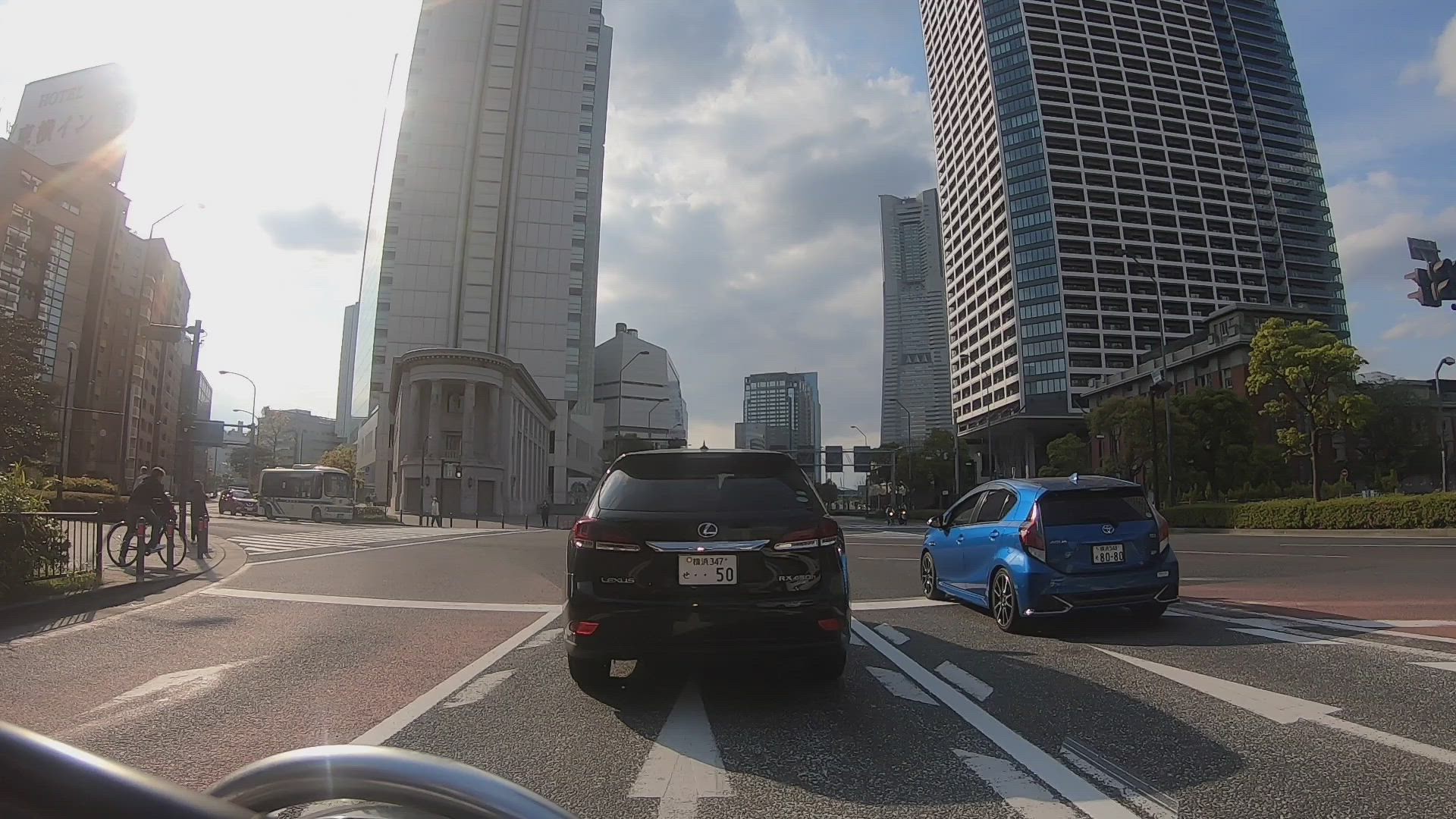A street view photograph taken from within a vehicle captures a bustling cityscape. The bottom frame reveals a silver steering wheel, indicating the driver's perspective. Centered in the image, a white forward-facing arrow is painted on the road, leading directly ahead. Positioned slightly to the left, a black SUV occupies the nearest lane while a blue two-door car is visible further ahead on the right.

The scene is framed by towering skyscrapers against a clear, blue sky. On the right, a sizable building with numerous windows suggests an apartment complex. To the left, a taller, narrower structure stands prominently. The road features directional arrows, including a white forward arrow on the right and a left-turn arrow on the left. Additional buildings rise in the distance, completing this vivid urban vista.